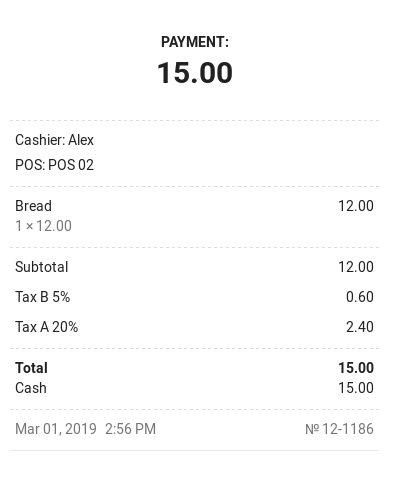The image is a screenshot of a receipt, featuring a white background. Centered at the top, in bold black capital letters, is the word "PAYMENT". Directly below, in very large numerals, is the amount "15.00", although there is no accompanying currency symbol, presumably indicating $15.00.

On the left side of the receipt, in a smaller font, it states "Cashier: Alex". Below this, in capital letters, is "POS", which likely stands for Point of Sale, followed by "POS 02".

A thin gray line separates this section from the itemized details below. The purchased item listed is "Bread" on the left, with the corresponding price of "$12" on the right side. Underneath this line item, it states "1 x 12", indicating one unit of bread priced at $12.

The subtotal is noted as $12.00. The receipt details two taxes: "Tax A 5%" which amounts to $0.60, and "Tax A 20%" which amounts to $2.40. 

At the bottom of the receipt, the total amount is shown as $15.00. It indicates that the payment was made in cash, specifically "$15".

Additionally, in the bottom left corner, the date and time are displayed as "March 1st, 2019, 2:56 PM". In the lower right corner, an identification number is printed: "No. 012-1186".